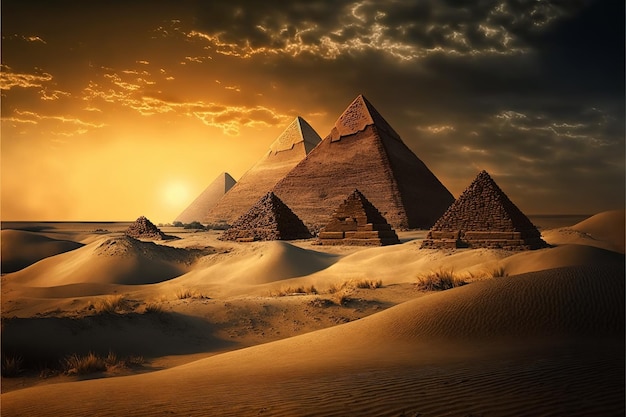This computer-animated image showcases a desert landscape illuminated by the golden hues of either early morning or late evening light, suggesting that the sun is either rising or setting. Dominated by shades of tan and brown characteristic of sandy terrains, the scene features a total of six, possibly seven, pyramids arranged in a staggered height sequence.

In the backdrop, the largest and darkest brown pyramid stands prominently, with a slightly smaller and lighter brown pyramid adjacent to it. Further in the distance, a light tan-colored pyramid can be seen, adding depth to the composition. 

In the foreground, three more pyramids continue the gradient. Starting from a very dark brown pyramid, the series progresses to a medium brown pyramid, followed by another dark brown pyramid, creating a rhythmic pattern across the image. Off to the leftmost edge, there is a hint of an additional pyramid, partially obscured and adding mystery to the expansive desert vista.

Above, the sky is dotted with wisps of clouds, enhancing the serene yet majestic atmosphere of this ancient-inspired setting.